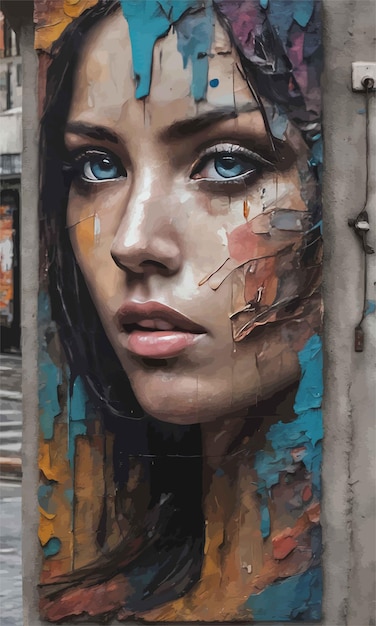This artwork is a vertically oriented painting, likely adorning the side of a building, depicting a stunningly realistic portrait of a woman who appears to be of Caucasian or possibly Hispanic descent. The woman is characterized by her deep blue eyes, dark eyebrows, and pink, parted lips. Her long, dark brown hair cascades down to her shoulders, covering her right ear, while her left ear is obscured by the edge of the composition. She gazes slightly off into the distance.

The painting artistically integrates a vivid palette of blues, oranges, yellows, and reds, which are smeared and layered across her forehead, cheeks, and neck, giving the piece a stylized and dynamic texture. The use of both soft brushes and a palette knife (or a similar hard tool) is evident, creating a blend of smooth and smudged effects throughout the portrait. The vibrant colors and textural elements add a unique depth, making the woman's face emerge strikingly from the abstract background.